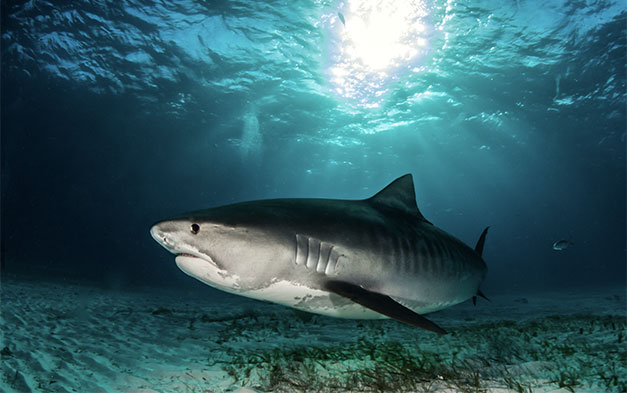In this detailed underwater photograph, a large tiger shark commands the scene as it swims near the sandy seafloor of the ocean. The background is a clear, deep, dark blue, which accentuates the various elements in the image. The shark, moving towards the camera but slightly turning to the left, displays a striking color gradient from its dark gray top, through lighter gray sides, to its white underside. The shark's side profile is visible, showcasing its gills, a single eye, and its slightly open mouth that reveals rows of jagged teeth. Vertical stripes, characteristic of its species, adorn its body, beginning to fade with maturity. Adding to the visual richness, patches of green seaweed grow sporadically on the sandy bottom. Above, a white light source, presumably the sun, casts bright rays into the underwater scene, highlighting different elements and creating interplay between light and shadow. The clean, clear water provides an unfiltered view of the majestic predator and the serene, yet vibrant underwater environment.